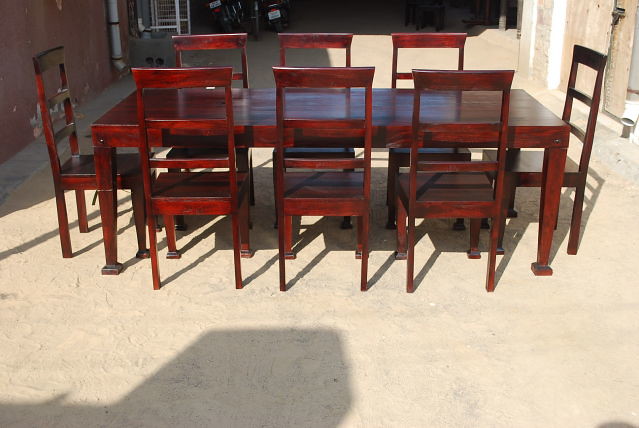The image features a dark reddish-brown wooden table, possibly cherry or burnished wood, situated outdoors. The table is long and rectangular, with eight matching wooden chairs—three on each side and one at each end. Each chair has a backrest consisting of two vertical wooden pieces with three open slots and a flat wooden seat. The setup is positioned on a concrete ground, which has a mix of shadows predominantly on the left-hand side and a sandy or tan appearance. 

Behind the table, two motorcycles are visible parked in front of a building that has dark gray sides and a portion of a pinkish wall with a white gutter and some gray elements held on with red. In the far distance, another wooden wall is barely visible, along with an open space that isn't clearly defined. The entire scene appears to be a backyard or an outdoor area adjacent to a garage, characterized by a serene yet functional ambiance.